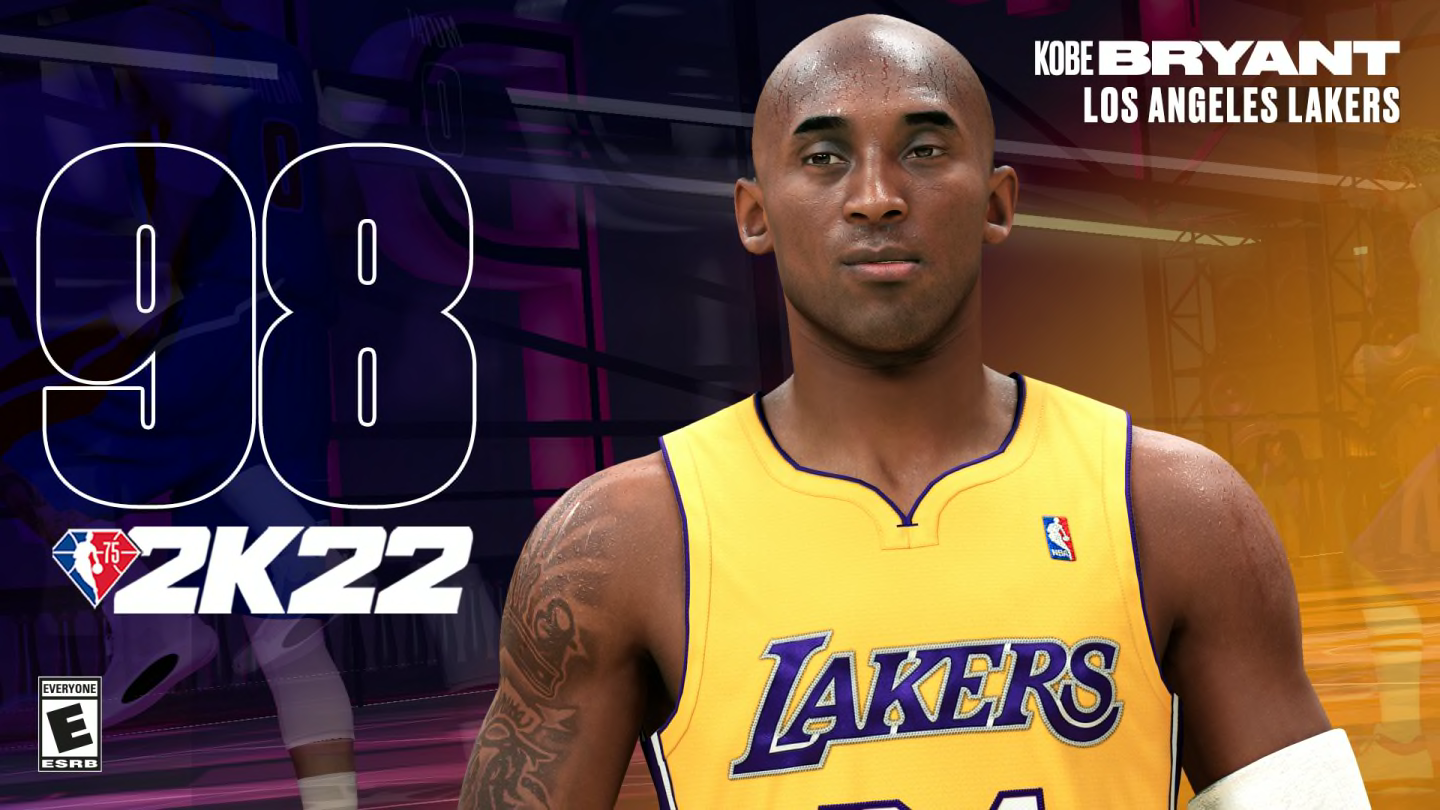This is a detailed photograph featuring Kobe Bryant of the Los Angeles Lakers. The image shows him from the mid-chest up, wearing a sleeveless yellow Lakers jersey emblazoned with "LAKERS" in purple. Tattooed in black ink, his right arm is quite distinct, and his bald head stands out against the vibrant background. Kobe, an African-American, is gazing towards the bottom left corner of the image.

The left side of the background is purple, while the right side transitions to a golden color. Overlaying the left side of the image is the white-outlined number "98" and on the right, "2K22" is written in solid white, all in capital letters. Below these numbers, positioned in a small white rectangle, is the ESRB rating "E for Everyone."

In the upper right corner of the image, "KOBE BRYANT LOS ANGELES LAKERS" is displayed in all caps, white font. An NBA logo in blue, white, and red is located on the upper left side of Kobe's jersey. The positioning and color contrasts in the composition highlight both the player and the text, creating a captivating visual tribute to the basketball legend.